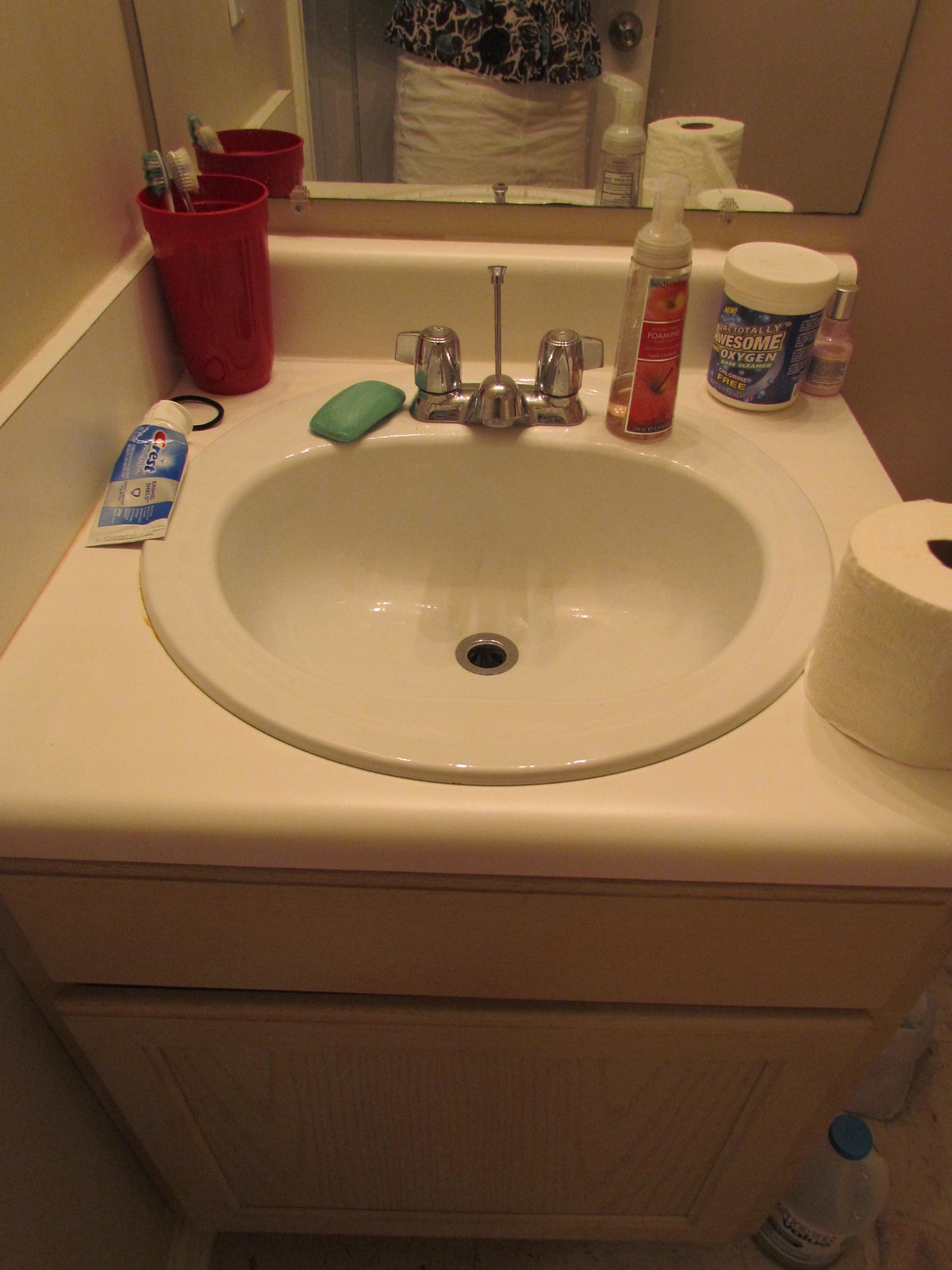The image depicts a bathroom sink and counter. Reflected in the mirror is an individual wearing a white skirt or pants paired with a dark, patterned shirt. The counter is adorned with various items, including a roll of toilet paper and a product labeled "Totally Awesome Oxygen," the rest of which is unreadable and likely related to bathroom use. 

Adjacent to these items is an indistinct pink object situated near the corner of the sink. A nearly finished bottle of foaming hand soap, seemingly apple-scented, displaying an apple on the label, is also present. Additionally, there is a blue hand soap and a tube of Crest toothpaste positioned to the very left of the sink. 

A hairband is laid out on the counter, alongside a tall red cup in the top left corner, containing two toothbrushes. The sink itself is a pearly white hue, matching the slightly cream-colored counter. The structure supporting the sink appears to be constructed of light-colored wood. A glimpse of a cleaning detergent bottle is visible on the floor to the right, though the exact floor details remain obscure.